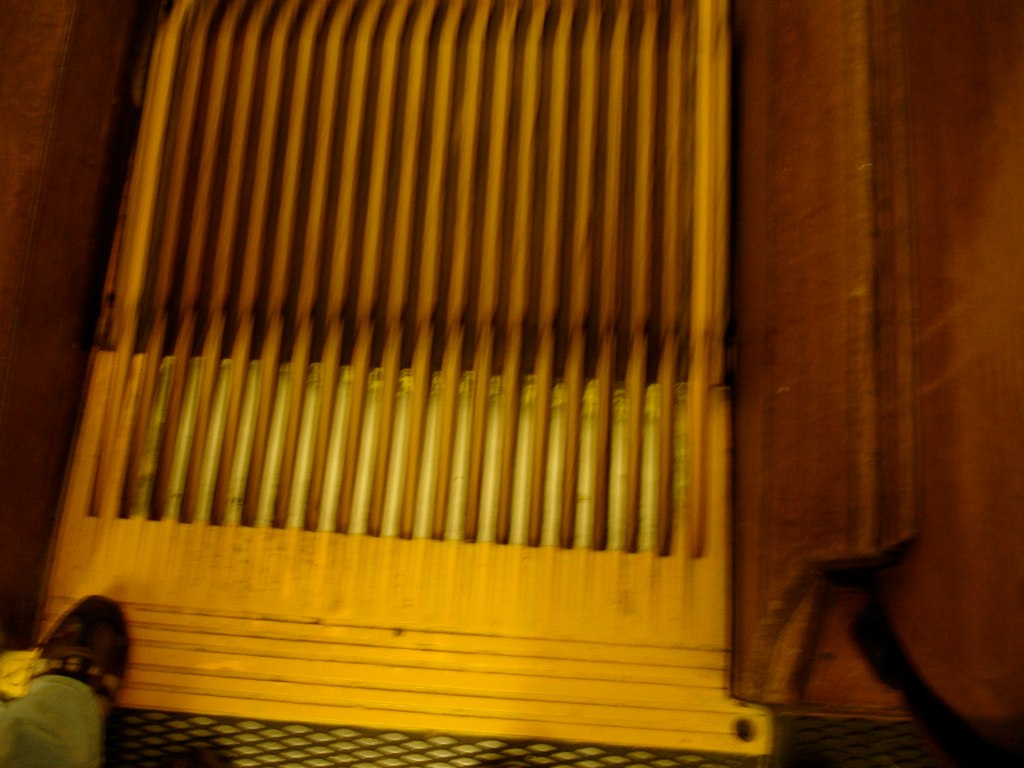The image captures a downward view at the top of an escalator. In the bottom left corner, a person's foot in a shoe extends from a pair of blue jeans, poised right before stepping onto the moving stair. The left and right sides of the image are framed by wooden structures showing some scratch marks, adding to the worn aesthetic. A golden metallic feature runs vertically in the centered upper area, reminiscent of organ pipes but identified as the escalator's comb plate with vertical gaps between each bar. Directly behind the foot is a metal grate, leading up to the golden structure where the moving stairs and the comb plate meet. The detail includes a significant bolt securing the plate visible on the right side, adding to a highly textured, slightly blurred, complex visual of intersecting materials and structures.